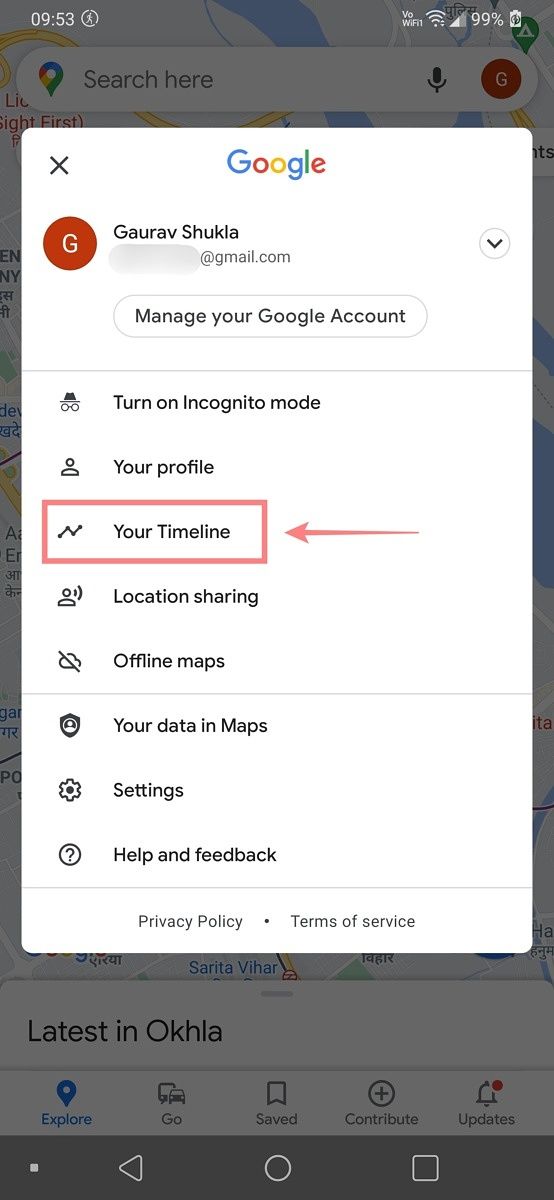Here is a cleaned-up and detailed caption for the image described:

---

This color photograph displays a mobile phone screen featuring a pop-up box overlaying the interface. In the upper left corner of the screen, the time reads 09:35, while the upper right corner displays white text indicating phone icons and a 99% battery level. The background, somewhat greyed out, shows a Google search bar.

The pop-up box in the foreground has a white background and is adorned with a multi-colored Google logo centered at the top. To the left of the logo is a small 'X' for closing the pop-up, while to the right, "Neil Perth" is displayed. Below this, a red circled 'G' icon appears next to the text "Garebov Shula," with part of an email address ending in "@gmail.com" partially obscured and a downward arrow to the right of it.

A curved rectangle below this text prompts the user to "Manage your Google Account." Underneath, a thin grey horizontal line separates this section from a list of options, each accompanied by small icons: "Turn on Incognito mode," "Your profile," and "Your timeline," these three being outlined with a red rectangular border, highlighted further by a red arrow pointing at them from the right side.

Following this, additional options include "Location sharing" and "Offline maps," separated by another thin grey line. Further options such as "Your data in Maps," "Settings," and "Help & feedback" are listed, followed by yet another thin horizontal line.

At the bottom, in grey text, lie links to the "Privacy policy" and "Terms of service." The very bottom portion of the screen reveals the standard mobile navigation bar with icons for back, home, and a square button.

---

This detailed caption highlights the visual elements and layout of the mobile phone screen and its contents.